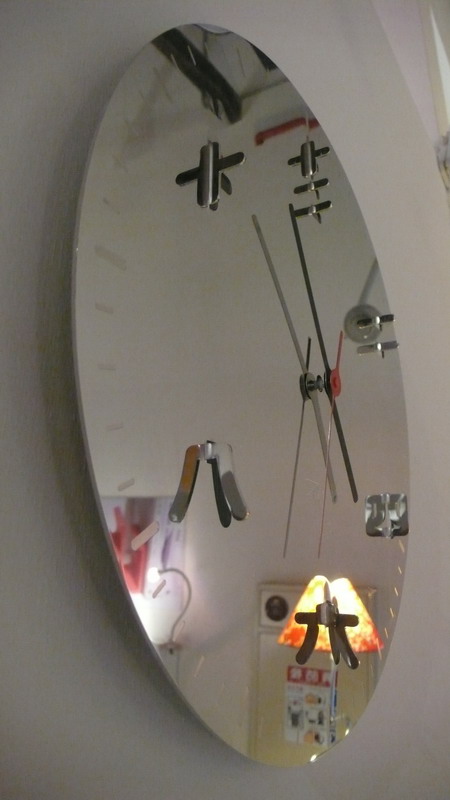This angled, close-up photograph captures a unique circular clock hanging on a white wall. The clock's face is a mirror, reflecting its surroundings: in the bottom right corner, there is a lamp and a poster with some indistinct work-related text, while in the bottom left, another lamp and poster are visible. The clock itself does not have traditional numbers; instead, it features metal prongs at the positions where numbers would typically be. The timepiece includes two thin hands: a long black hour hand and a slightly longer, thin red minute hand, which are mirrored on the reflective clock face. The clock is set to approximately 3:55, with the second hand positioned at 35 seconds. The faint lines around the clock and various mechanical-looking metal pieces contribute to its distinctive aesthetic.